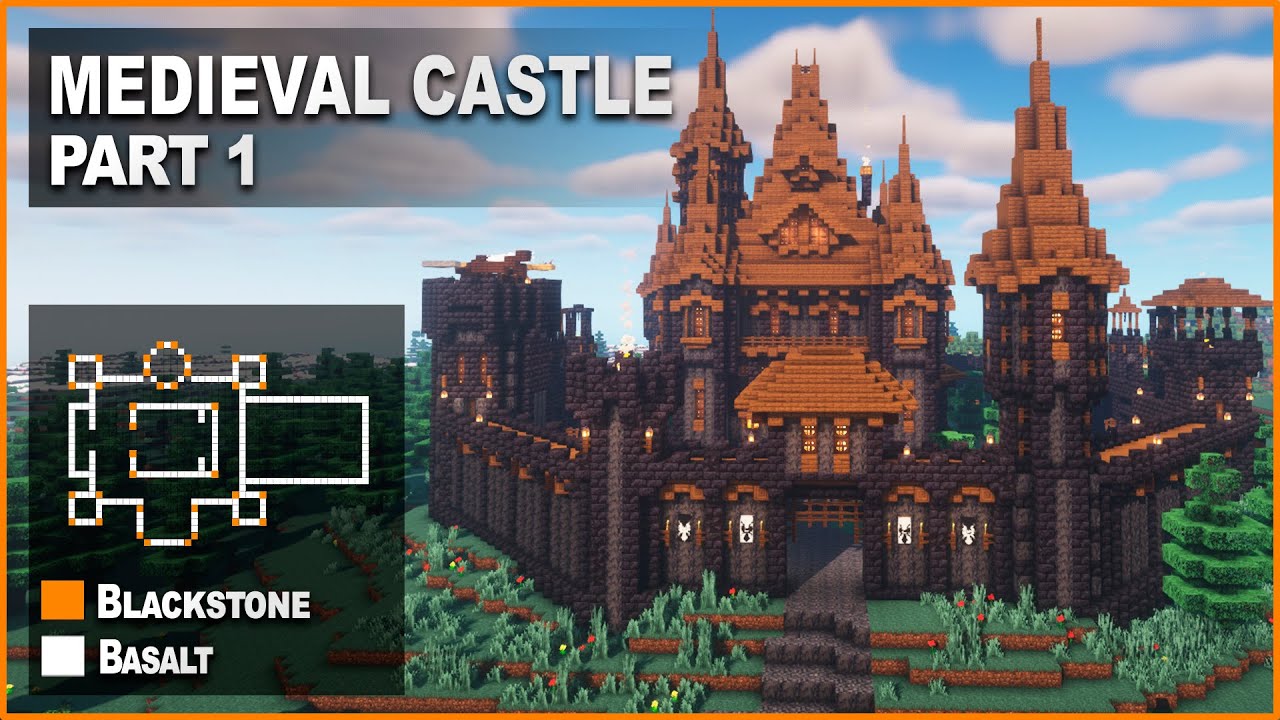The image serves as a thumbnail or banner for a step-by-step how-to guide on building a structure in the popular video game, Minecraft. Framed by a thin orange border, the rectangular image features vibrant, Bloxy-like textures typical of the game. In the foreground, a large black castle with a brown roof dominates the scene, constructed from distinctive 3D blocks. The setting is outdoors, with lush green trees and a clear blue sky interspersed with fluffy clouds.

In the top left corner of the image, a semi-transparent rectangle with white text reads "Medieval Castle Part 1." In the bottom left corner, another semi-transparent black square contains the words "Blackstone Basalt," along with an intricate white floor plan of the building. This detailed image, reminiscent of a Lego design, invites viewers to embark on the first part of an exciting medieval castle-building journey.